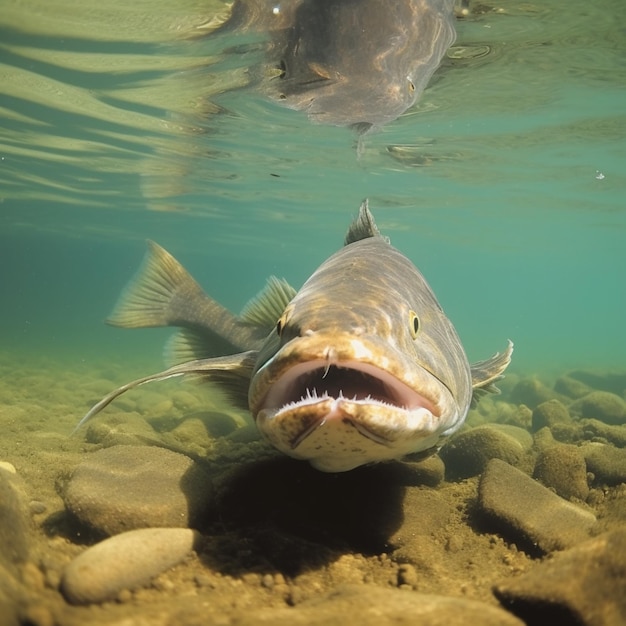The image depicts a large fish, possibly a catfish or carp, swimming in shallow, muddy water. The fish is facing the camera with its mouth partially open, showcasing sharp, small teeth. Its eyes are yellow with black pupils, somewhat bulging from the sides of its grey, brown, and white mottled body. Just below the water's surface, near the rocks and sand-covered bottom, the fish's dorsal fin almost touches the surface. The water appears polluted and hazy, giving a blue and dirty appearance to the background, while round rocks are clearly visible in the foreground, covered in brown dirt. Reflections and rippling patterns on the surface of the water highlight the fish's silhouette. There is also another fish partially visible near the surface, with only its underbelly discernible.